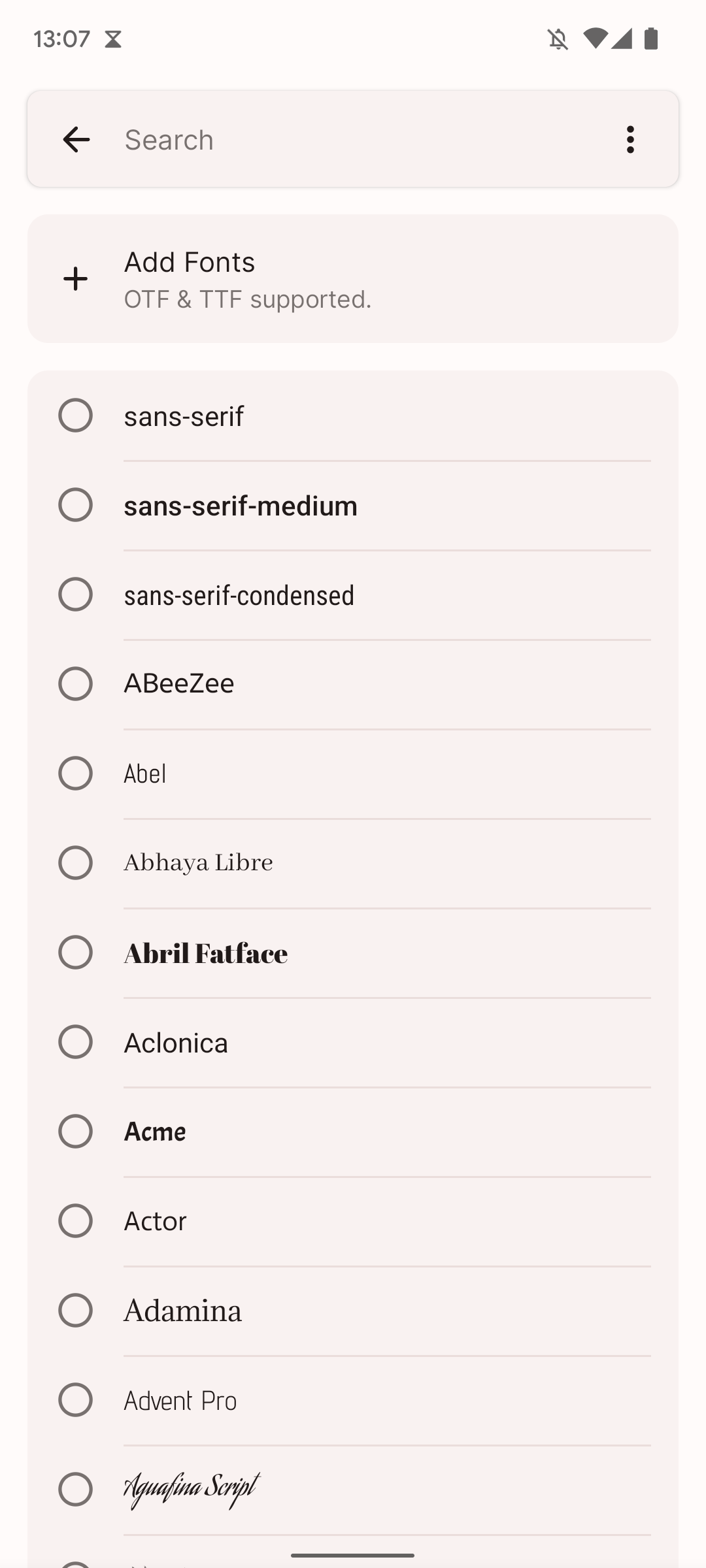This is a detailed screenshot of a smartphone's interface, displaying a time of 13:07 at the top, flanked by icons indicating a strong internet connection and a full battery charge. Below the status bar is a gray search bar with an arrow pointing to the left and a menu icon of three dots to the right. 

The subsequent section, slightly tinted with a pink hue, features a box with a plus sign on the left and the text "Add Fonts". Beneath this, it states "OTF & TTF supported". Following this, there is an extensive, scrollable list of various font types, each accompanied by an unhighlighted circle on its left.

The list begins with "Sans Serif," followed by "Sans Serif Medium," which appears slightly bolder. Next is "Sans Serif Condensed," notable for its smaller and tightly spaced appearance. Further down, a series of font names include:

- "ABC (capital letters), abc (small letters), and ABeeZee"
- "ABEL" in light black, with a small, understated look
- "ABHAYA Libre"
- "ABRIL Fatface," distinguishable by its thicker, black font
- "Aclonica"
- "Acme," a smaller-sized, darker black font
- "Actor"
- "ADAMINA," a somewhat larger font in a medium black shade
- "Advent Pro," characterized by a very thin, light black font
- "Aquafina Script," a dark black cursive style

Each font name is precisely noted in different styles, offering the user a variety of options for text personalization.